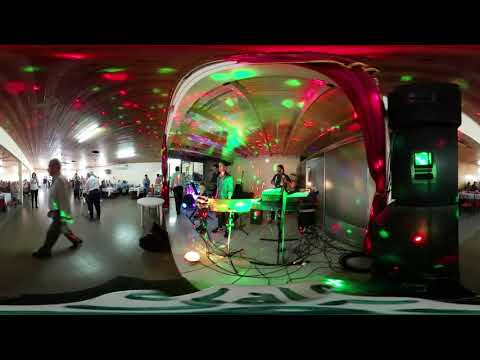The image depicts the inside of a large indoor space, possibly a convention center or shopping mall, with a distorted, fisheye effect creating a curved appearance. Central to the scene is a clear bubble-like enclosure, housing a musical band complete with visible instruments, keyboard stands, and chords. The bubble has a curtain on its left side, and inside, the ceiling displays vibrant red and green strobe lights that resemble those from a disco ball. The space outside the bubble features smooth grey flooring, brown roofing, and scattered tables and chairs where people are sitting or walking around, many in white shirts and black pants. To the right of the bubble is a machine resembling an ATM with green and red lights. At the bottom of the image, there is a green and white sign, partially obscured by horizontal black strips at both the top and bottom of the photo. The overall atmosphere is lively and colorful, characterized by the dynamic lighting and bustling crowd.